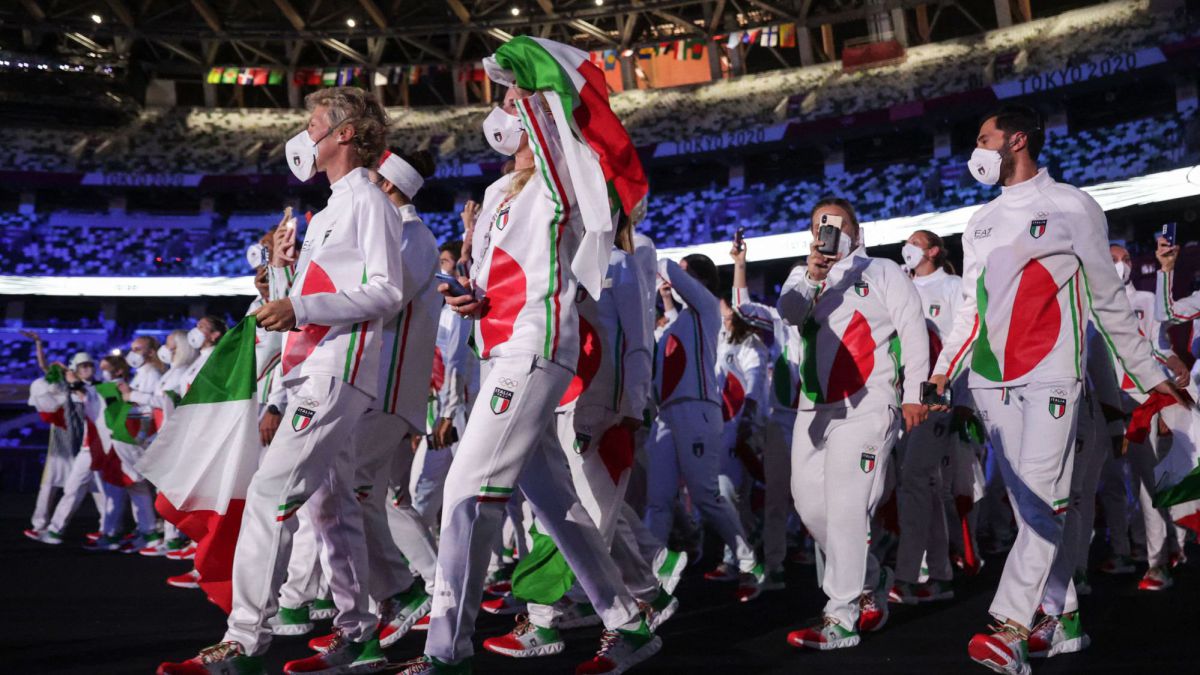The image displays a vibrant scene of what appears to be the Italian Olympic team making their grand entrance during the opening ceremony of the Tokyo 2020 Olympics. The athletes, dressed in matching white track suits adorned with the Italian flag's colors—green, white, and red—are also sporting coordinated shoes in the same color scheme. Each member wears a COVID-19 protective mask, suggesting the image was taken during the pandemic. Some athletes carry Italian flags, while a few capture the moment on their phones.

They are walking into a large stadium with a partially covered, open roof. The stadium's grandstands are filled with a cheering crowd, their faces illuminated by a cool purple light, contrasting with the more focused stadium lights that highlight the athletes. A scoreboard or a sign in the background displays "Tokyo 2020," affirming the event's setting. This close-up view captures the expansive nature of the team, which seems to comprise between 50 to 100 athletes, filling the depth and breadth of the image. The entire scene is imbued with a sense of excitement and national pride as the athletes march forward, united in their striking tricolor attire.